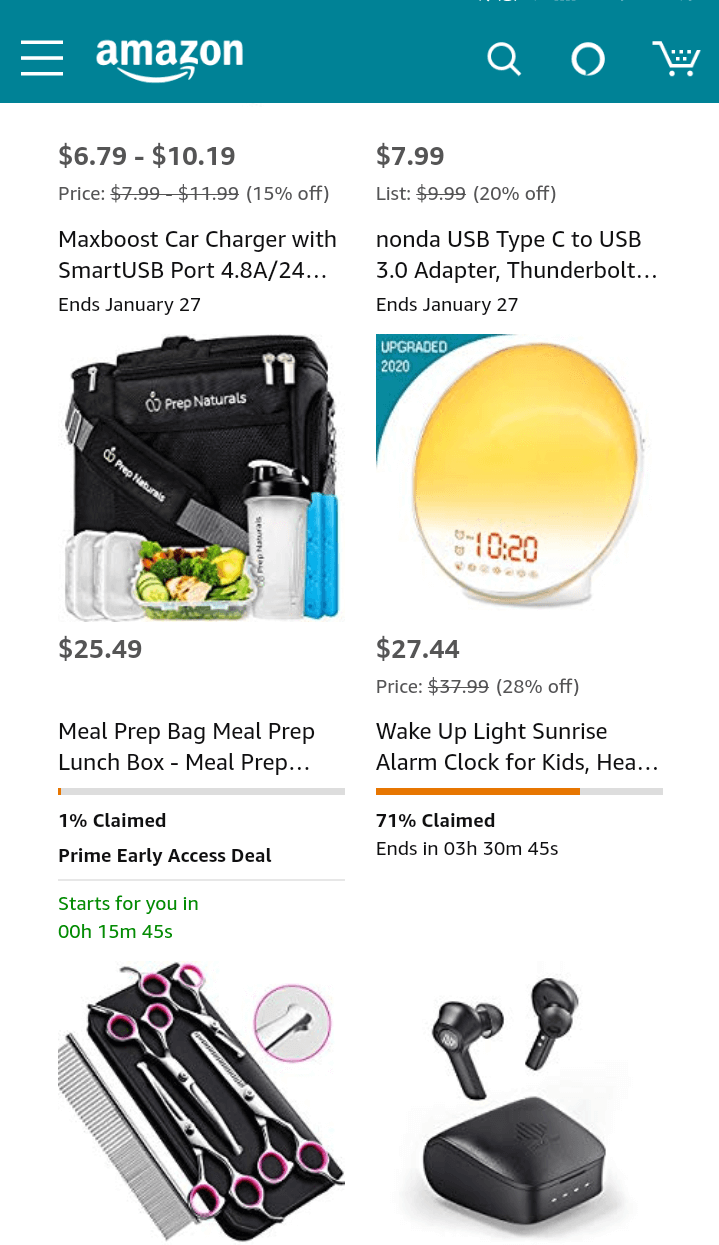The image captures the interface of the Amazon app. At the top of the screen, the iconic Amazon logo is prominently displayed in white text, with the trademark smile connecting the 'A' to the 'Z', also rendered in white. Adjacent to the logo, there is a magnifying glass icon representing the search function, a circular symbol, and a shopping cart icon, all set against a blue background.

Below the header, a variety of product listings are showcased, each featuring detailed information. 

1. The first product is a Max Boost Car Charger with a Smart USB Port, priced between $6.79 to $10.19. This listing includes an image of the product, which appears to be a car charger, and mentions an end date of January 27th. 

2. Another highlighted item is a Prep Naturals meal prep bag, priced at $25.49. The listing description reads "Meal prep bag, meal prep lunch box, 1% claimed," indicating it is part of a Prime Early Access Deal.

3. The next featured product is a Wake Up Light Sunrise Alarm Clock for kids. The listing shows that 71% of this item has been claimed, with an orange progress bar illustrating the sales status. The deal for this item ends in 3 hours, 30 minutes, and 45 seconds, with a price of $27.44.

Further down the page, there are additional images of various products. One image depicts scissors or hair supplies in silver and pink, while another shows black earbuds alongside their carrying case, packaged beneath them.

Overall, the background of the product listings is white, with the details presented in black text, ensuring clarity and readability.